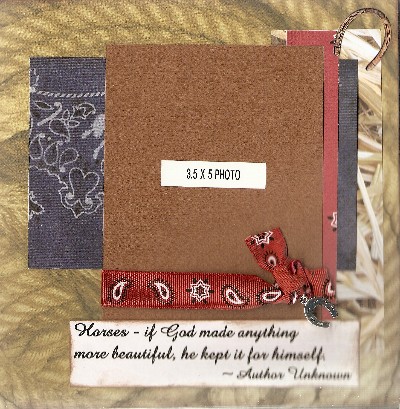The image presents a visually intricate and textured art project set against a background resembling a wheat-colored coiled rope or mat, giving it a rustic, cowboy-like aesthetic. The project is horizontally rectangular and features multiple layered elements, creating a collage effect. 

At the center is a brown square, possibly fabric or sandpaper, with a small white piece of paper taped to it, displaying the text "3.5 by 5 photo" in black lettering. This central element is wrapped with a red ribbon or fabric, resembling a dog collar. Beneath this are additional layers, including a piece of red fabric with intricate black and white designs and another blue fabric with white patterns.

On the right side, there appears to be a horseshoe ring, contributing to the Western theme. At the bottom of this arrangement is a white strip of paper containing a quote in a fancy script font: "Horses. If God made anything more beautiful, he kept it for himself. Author unknown."

The combination of textures and elements, from the coiled rope background to the layered fabrics and meaningful quote, gives the image depth and a rich narrative, evocative of a handcrafted homage to beauty and artistry.